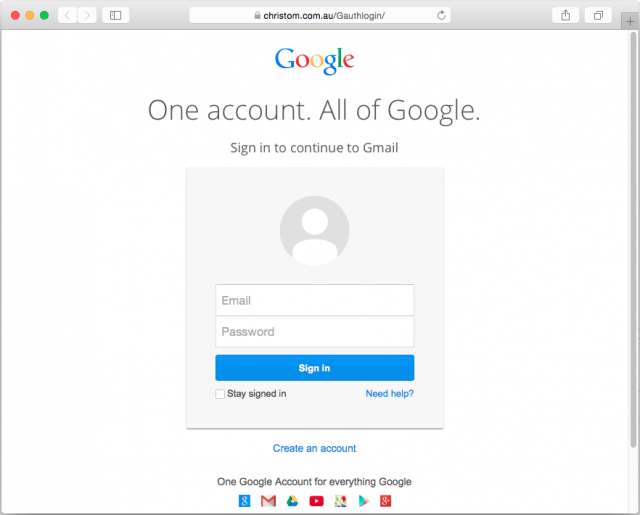The image depicts a login screen on an Apple product, likely an iMac, identifiable by the distinctive red, yellow, and green dots in the top left corner of the window. The background is entirely white with a blue title bar at the top, in which the web address "christom.com.au/gauthlogin/" is displayed. Central to the image is the familiar Google logo in its traditional colors, followed by the phrase "One account. All of Google." in gray font. Below this, the text reads "Sign in to continue to Gmail," prompting users to enter their email and password. Interactive options such as "Need help?" and "Create an account" (in blue font) are also present. Near the bottom, it states "One Google account for everything Google" in black font, accompanied by icons representing various Google services, including Gmail, Google Drive, YouTube, Google Maps, the Play Store, and the now-outdated Google Plus.